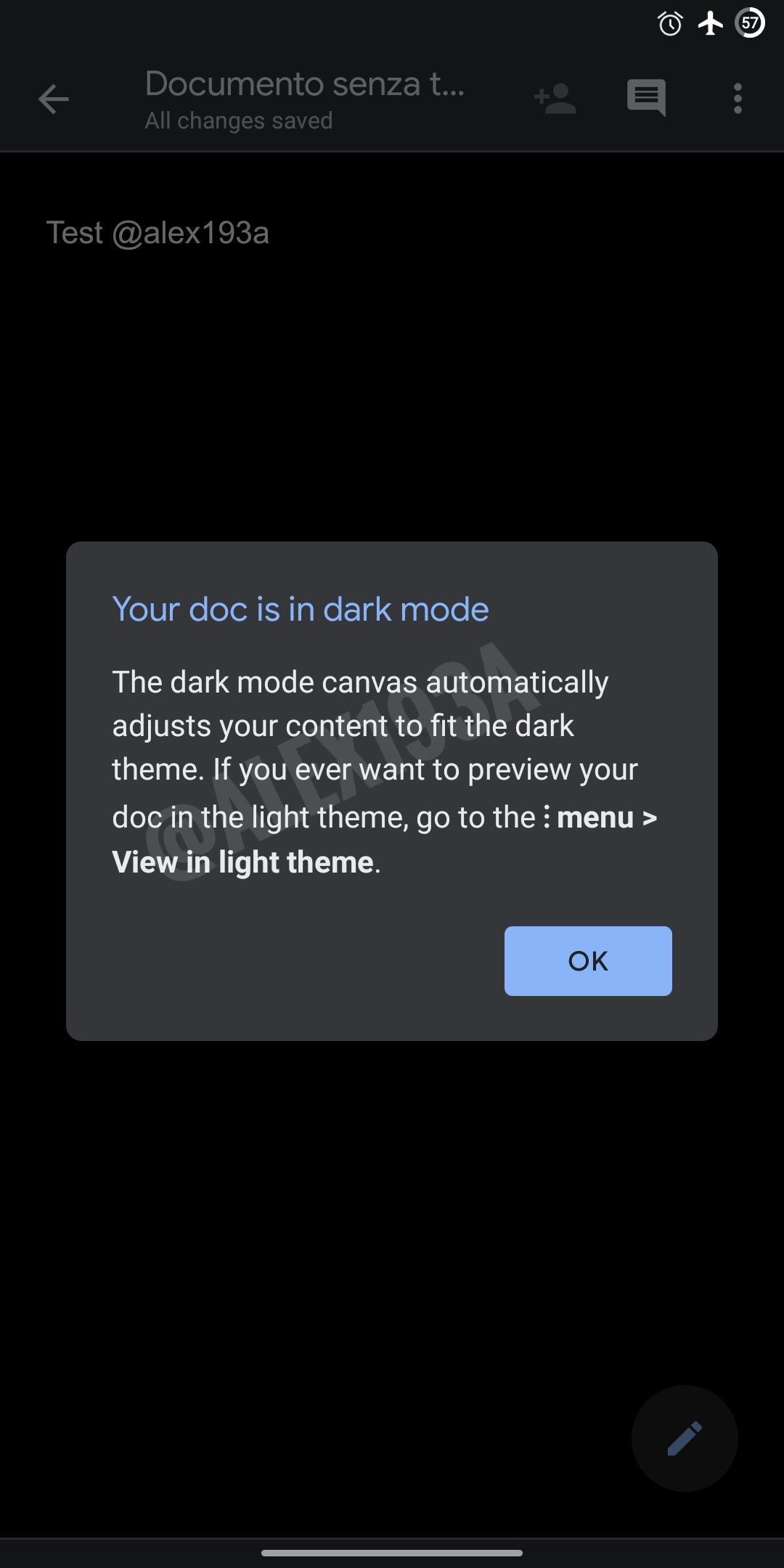The screenshot is from a mobile phone displaying an interface in dark mode, characterized by a black background. At the top of the screen, there is a charcoal gray rectangle. Within this top bar, on the upper right corner, three icons are visible: an alarm clock, an airplane, and a circle with the number '57' inside it.

Inside the charcoal gray bar, to the left, in gray font, the text "Documento Senza T..." is displayed. Directly below this, a message reads "All Changes Saved." On the left side of this bar is a gray arrow pointing left. Moving rightwards across the bar, there is a gray icon of a human silhouette with a small plus sign beside it, followed by a chat bubble icon and three vertical white dots.

Beneath this top bar, the remainder of the screen is black. At the top of this section, "Test at Alex 193A" is written in gray font. Below this, a pop-up menu is centered, with a gray background. At the top of this menu, the message "Your doc is in dark mode" appears in blue font. Further down, a description in white font explains, "The dark mode canvas automatically adjusts your content to fit the dark mode theme. If you ever want to preview your doc in the light theme, go to the: Menu > View in Light Theme."

Finally, the lower right corner of the pop-up features a purple square, containing the word "OK" in black font.